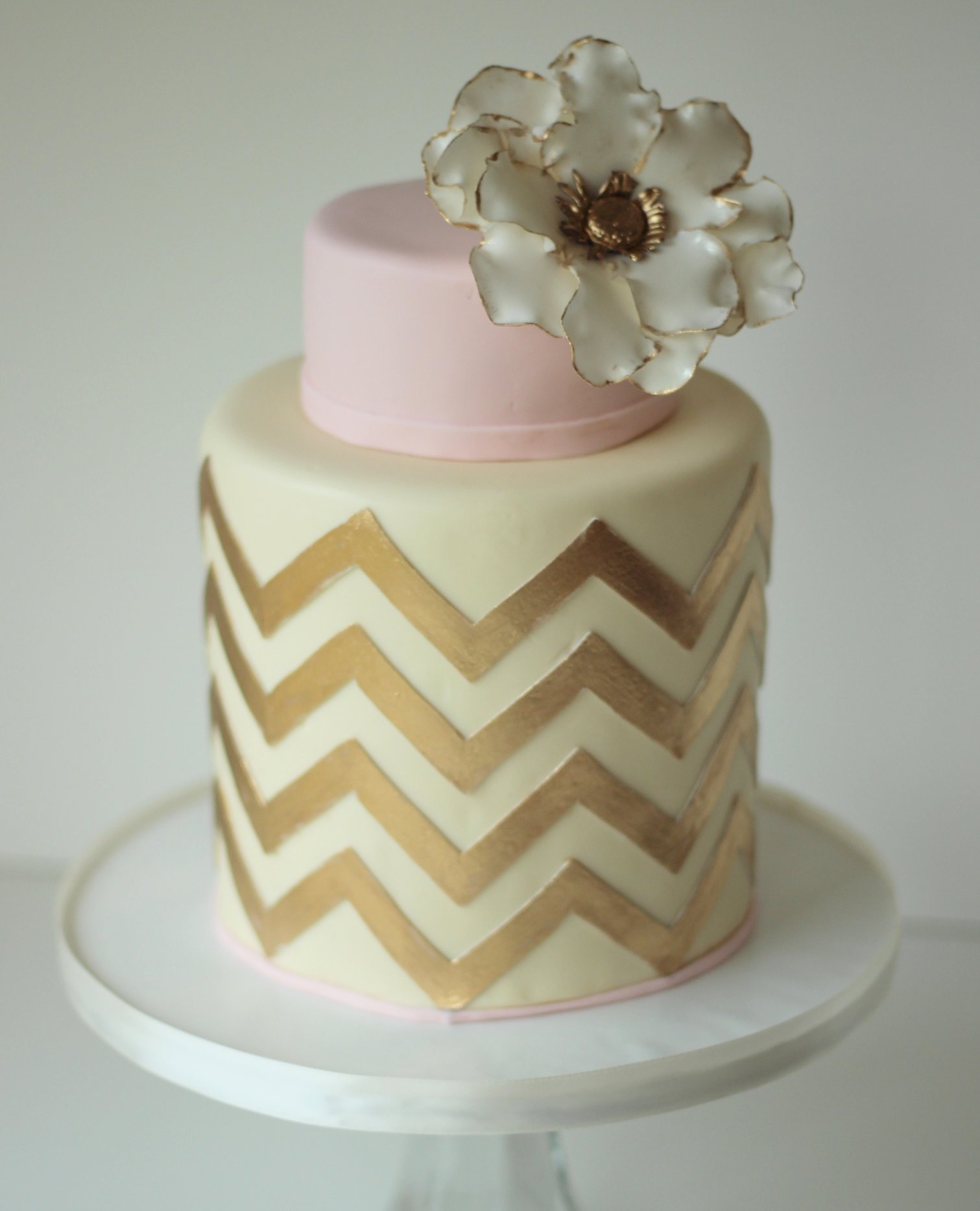This photograph features a beautifully detailed two-tiered cake placed on a small, white circular table with a transparent leg. The cake itself is predominantly cream-colored with a gold zig-zag pattern encircling the lower, taller cylindrical layer. Upon this layer sits a smaller, pink cylindrical layer adorned with a white and gold flower at the top right corner. In the center of this flower is a golden circle surrounded by dainty white leaves. The entire composition is elegantly centered against a white background, emphasizing the intricate and colorful details of the cake.